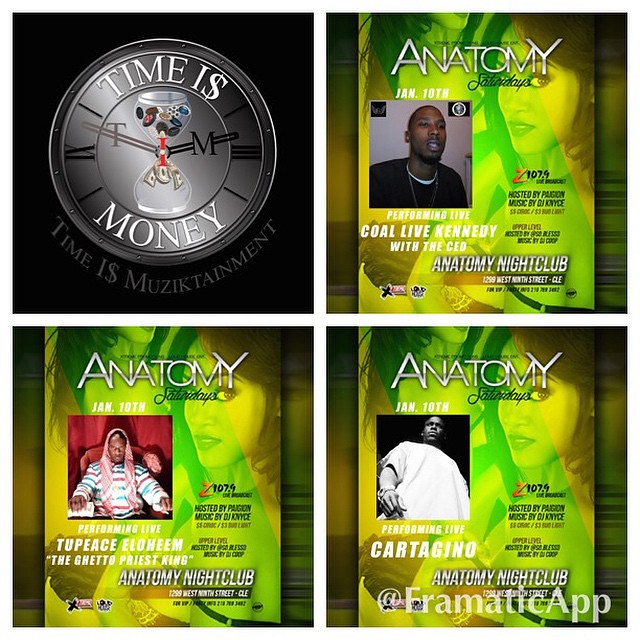The image is a promotional flyer divided into four sections, arranged in a windowpane grid layout that heavily emphasizes bold and contrasting colors such as yellow, green, silver, black, and white. The top left section features a grey clock on a black background with the phrases "Time is Money" and "Time is Music-tainment" displayed inside. This section stands out distinctively from the other three sections.

The remaining three sections share a consistent background showcasing two scantily dressed girls with the word "Anatomy" prominently displayed at the top in white font. Below this are photographs of different performers for each section. The first photograph highlights "Cole Live Kennedy with the CEO," the second advertises "Two Piece Elohim, the Ghetto Priest King," and the third features "Carter Gino." At the bottom of each of these sections, the name "Anatomy Nightclub" is clearly indicated, suggesting the venue for the performances.

Overall, the flyer aims to promote a nightclub event with multiple live performances, capturing the attention with vibrant colors and eye-catching graphic design, while providing essential details about the artists and location.